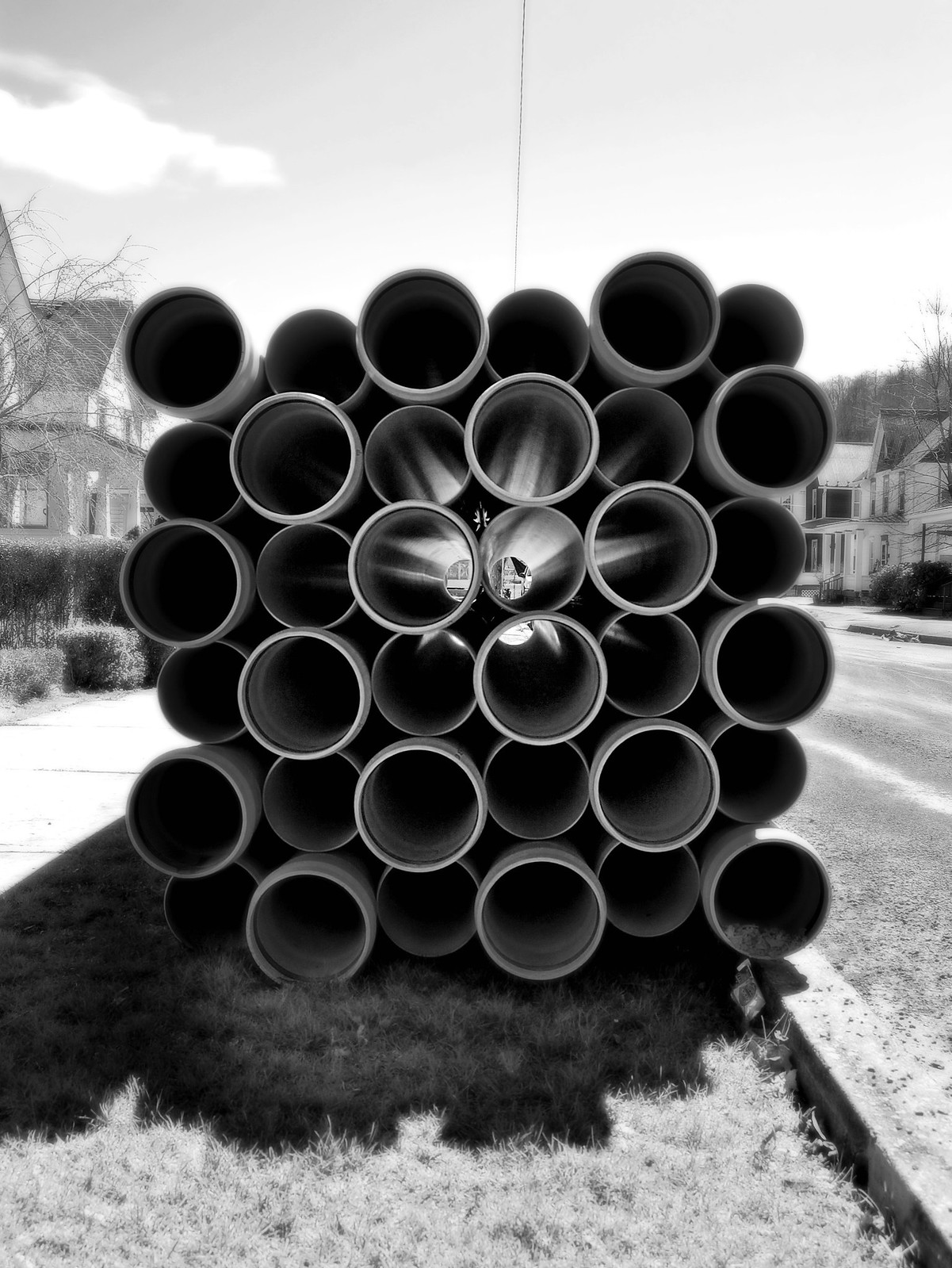This detailed grayscale painting depicts a suburban neighborhood scene under a gray sky adorned with a puffy white cloud on the left. The composition centers around a suburban street lined with a sidewalk and a small grassy verge. Row houses and trees stretch along both sides of the road, with additional bushes and branches visible on the left. Dominating the middle of the image is a substantial stack of black hollow pipes, numbering between 20 to 30, laid horizontally on the grassy plot. Notably, there is a faint, indistinct drawing or artistic marking inside the central pipes, adding a subtle layer of intrigue to the scene.